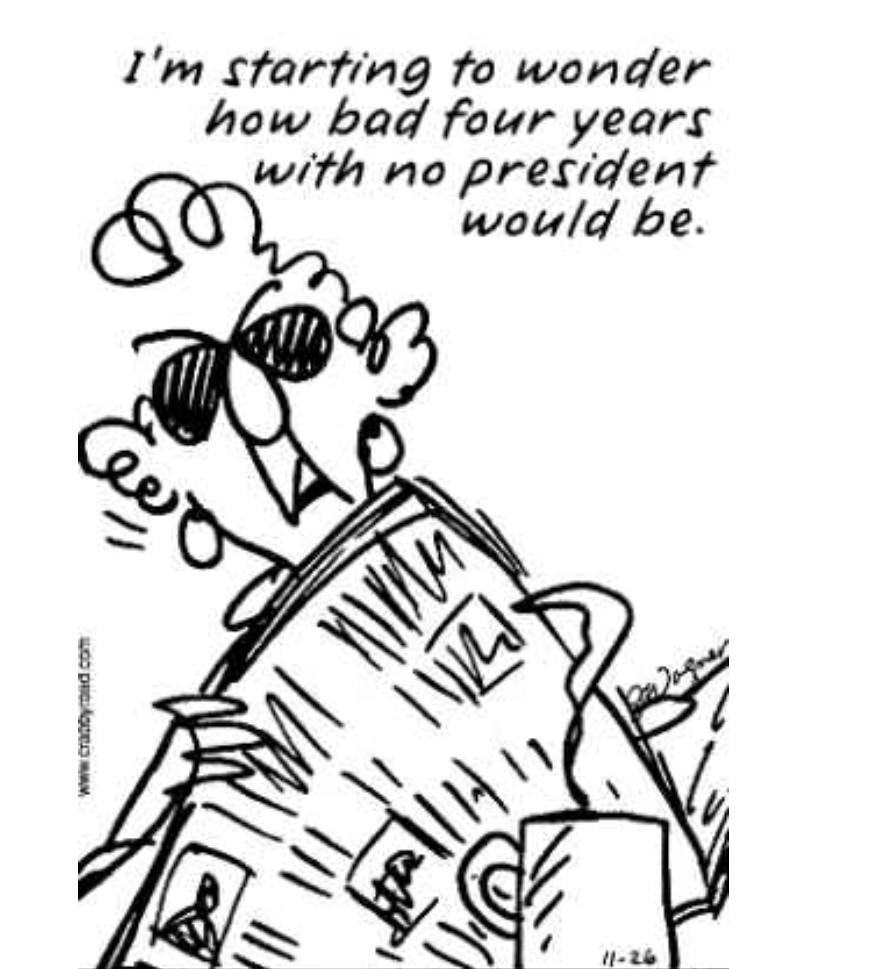This black and white cartoon features an elderly woman with dark, squiggly hair wearing black sunglasses and dangly, pearl-like earrings. She has a very grumpy, unpleasant expression and is holding a folded newspaper in one hand while a steaming cup of coffee or tea sits in front of her. The drawing is done in a rough, simple, and crude style with minimal details. In the background, there is a sketch of a sofa. Above her head, in blocky black lettering, the caption reads, "I'm starting to wonder how bad four years with no president would be," adding a touch of humor to the scene. Her head is slightly tilted to the left, further emphasizing her distressed and annoyed demeanor.